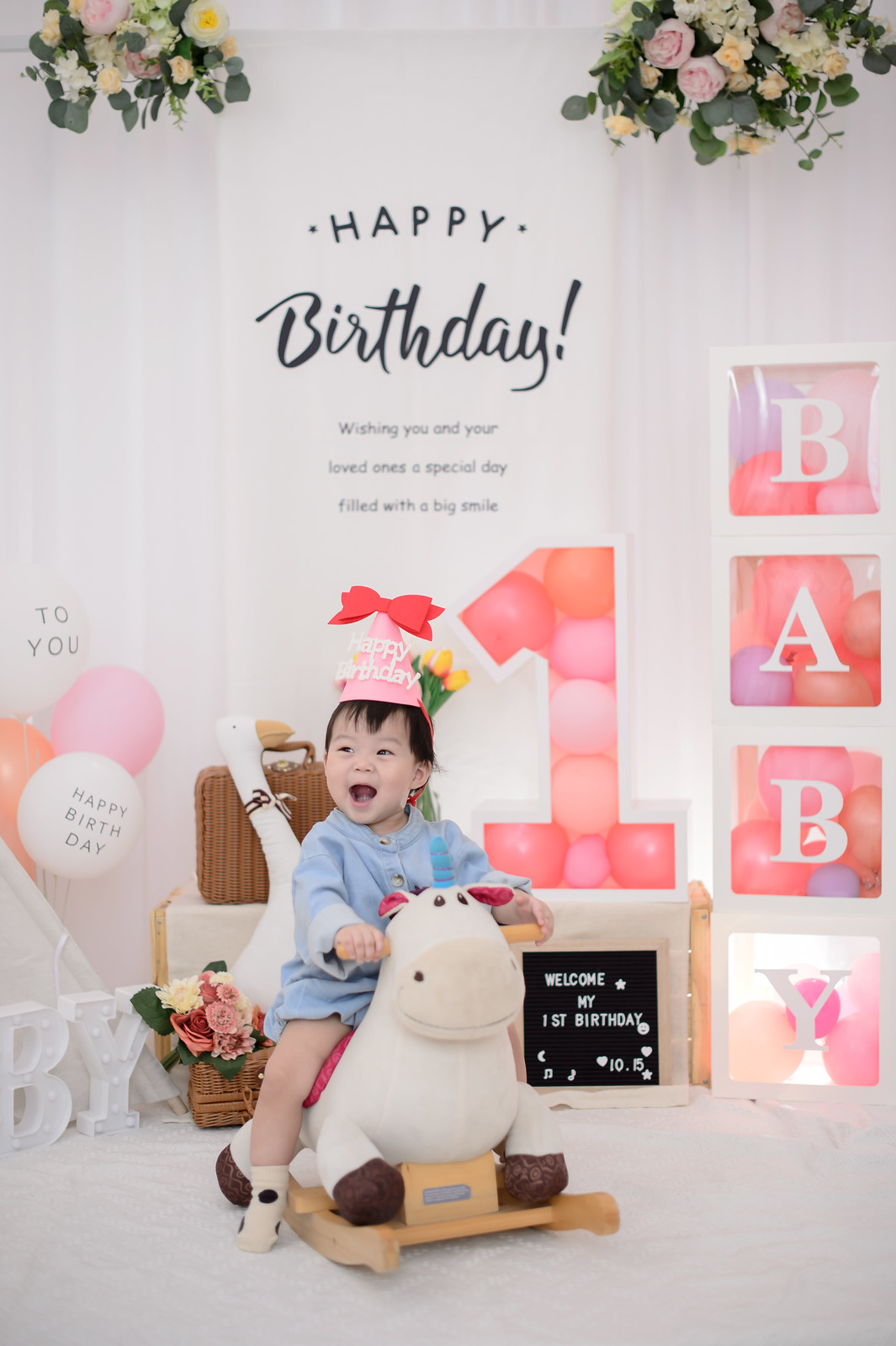This photograph captures an enchanting moment from a one-year-old’s birthday celebration. At the center of the image is an Asian child with light skin, dark hair, and a beaming smile, joyfully riding a stuffed animal that resembles a white hippopotamus acting as a rocking horse. The child is dressed in a light blue one-piece outfit paired with polka dot white socks, and a charming pink birthday hat adorned with a red bow that reads "Happy Birthday."

In the background, a white wall showcases festive decorations: a large, curved "HAPPY BIRTHDAY!" in black script, accompanied by additional smaller text, presumably conveying birthday wishes. To the right side of the wall is a large, festive numeral "1" in bright pink and orange, resembling a balloon splash. Also on the right, and vertically aligned, are transparent squares containing letters that spell out "BABY," filled with colorful balloons. On the left side, there are numerous white and pink balloons along with flowers and toys scattered on a pristine white laminate floor, adding to the celebratory ambiance. The upper corners feature graceful floral graphics, completing the whimsical and joyous scene.